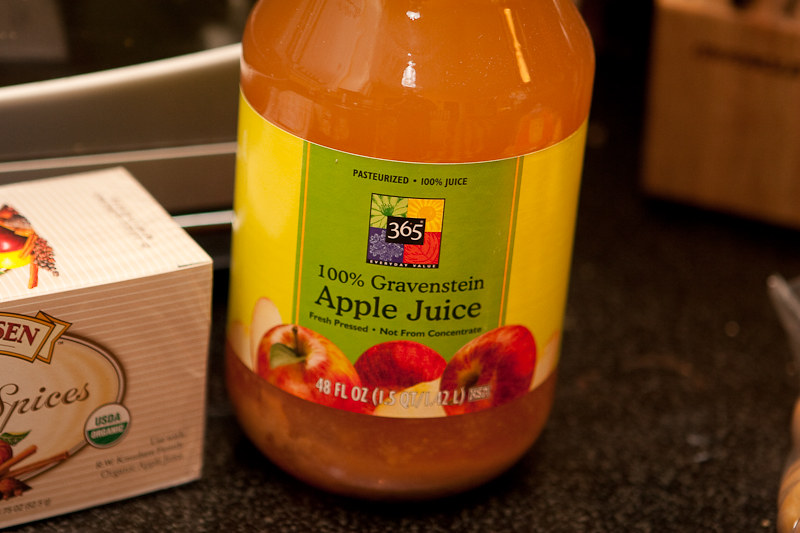This photograph captures a glass jar of pasteurized 100% Gravenstein apple juice prominently displayed on a black and white grainy countertop. The jar, filled with vibrant orange liquid, features a distinctive yellow and green label. The center of the label, green in color, boasts multiple lines of black text detailing "Pasteurized 100% Juice," "100% Gravenstein Apple Juice," "Fresh Pressed," and "Not from Concentrate." At the bottom of the label, illustrations of whole and sliced red apples are depicted, with their interiors showing a yellow or white hue, accompanied by white text indicating "48 FL OZ 1.5 QT 1.42 L." In the distance, a light brown wooden grain cabinet door is visible, adding a touch of warmth to the scene. The top of the jar is slightly cut off from the frame. Additionally, a box of tea adorned with a spice image and a USDA organic logo sits beside the jar on the countertop.